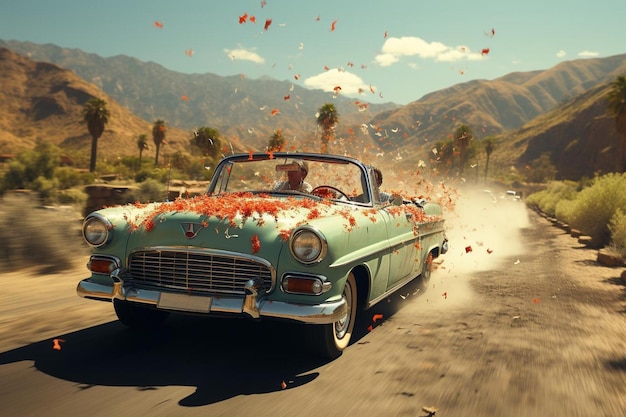This color photograph depicts a green 1950s American convertible speeding down a dirt road, kicking up dust beneath and behind it. The car, adorned with shiny aluminum bumpers and chrome trim, boasts two round headlights and elegant whitewall tires, as well as an open top. Seated in the front are two men, with one driving and the other as the passenger. The vehicle is splashed with vibrant red-orange flower petals, some of which are captured mid-air, seemingly flying off the car. The backdrop suggests a desert state like Arizona, marked by palm trees, sparse greenery to the sides, brown hills, and a blue sky dotted with white clouds. The scene conveys a sense of movement and adventure, with the natural landscape accentuating the vintage charm of the convertible.